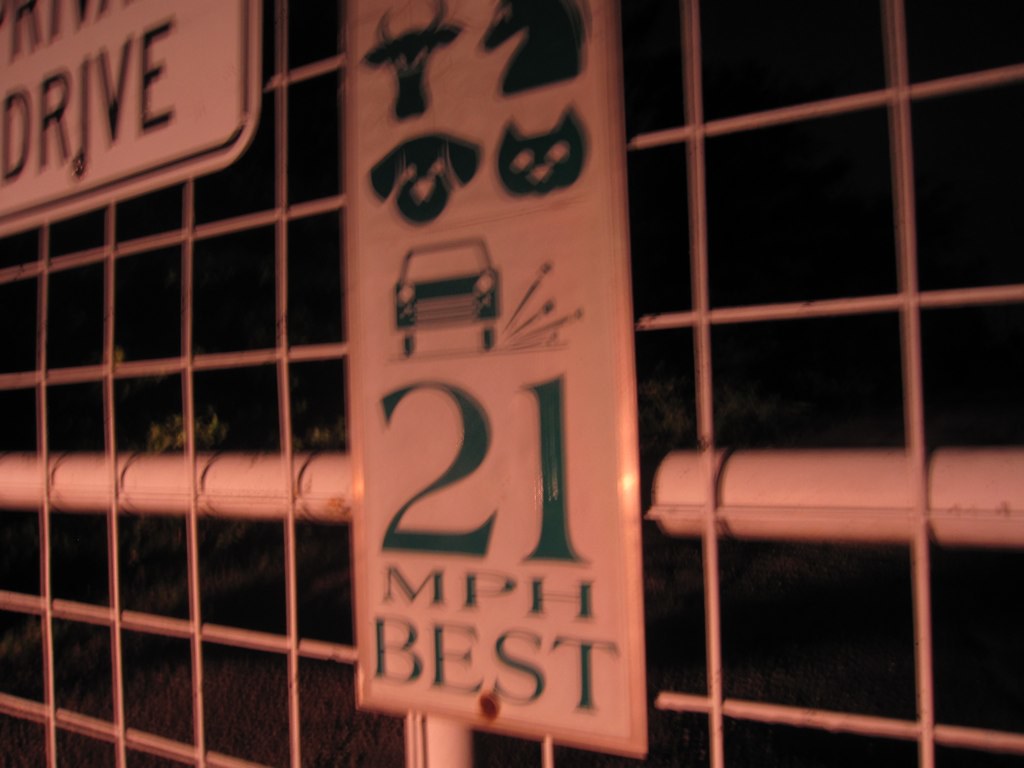**Descriptive Caption:**

The image showcases a vertical sign mounted on a white fence, set against a nighttime backdrop. The sign features a series of animal silhouettes running vertically down its length. At the very top, there is a silhouette of a cow's face with prominent horns. Directly below it to the right, a silhouette of a horse’s face and neck is depicted. Moving down, there is a silhouette of a dog's face followed by a cat's face. Beneath these animal images, the sign displays an illustration of a car with little sparks emanating from the right side of the vehicle. Below the car image, the text reads "21 MPH best," suggesting a recommended speed limit. In the top right corner of the sign, partially obscured text reads "Drive," with the rest cut off. The white fence behind the sign is complemented by a white pole and is partially obscured by a bush. The scene is dark, indicating that the photo was taken at night.